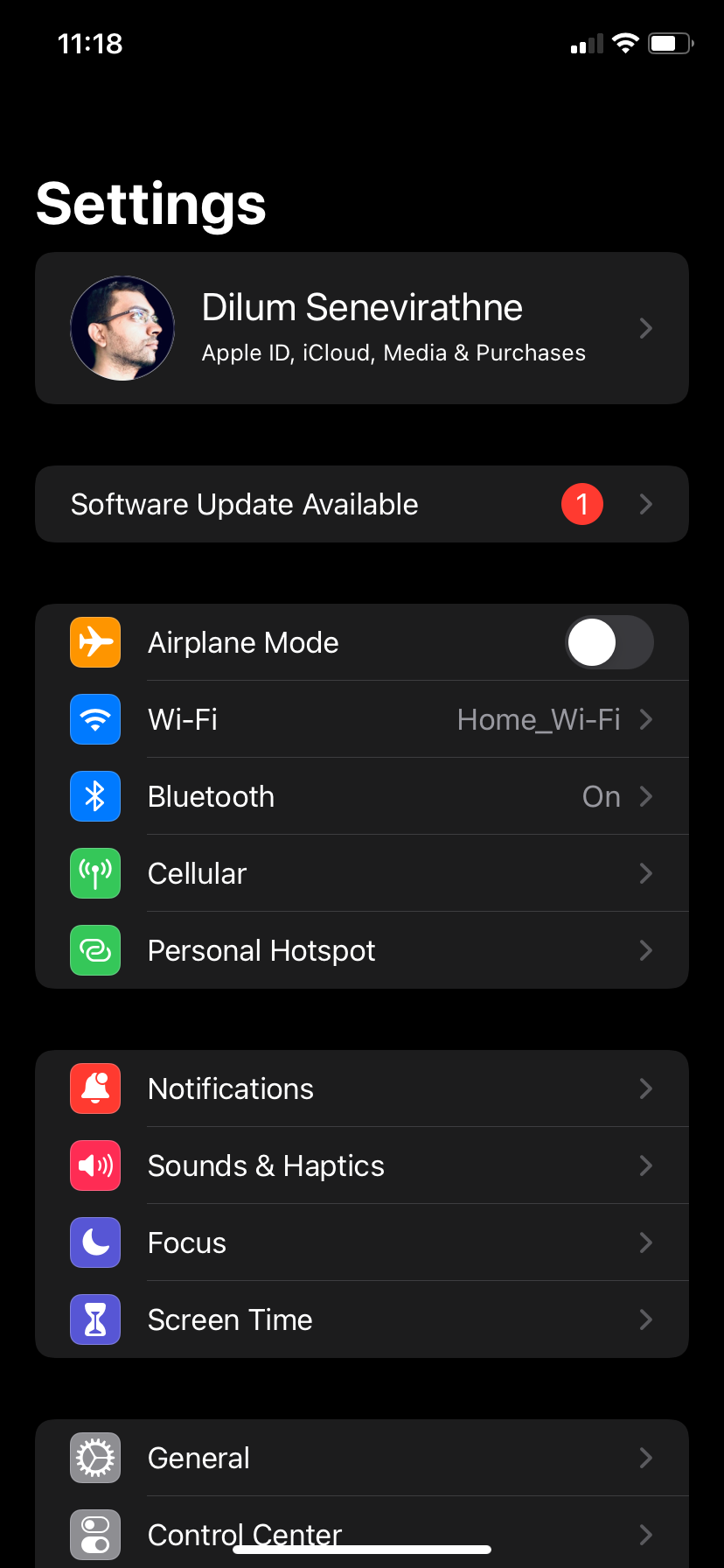The screenshot depicts the settings page on a phone, which appears to be an iPhone, contrary to initial impressions of it being an Android device. The display shows the time as 11:18, with signal strength at 2 out of 4 bars, Wi-Fi status indicating a strong connection, and the battery level at approximately 75%.

At the top of the settings page, there is a section for the user's profile, showing a profile picture of a Caucasian male with short brown hair and glasses, looking off to the right. The name displayed is "Dillon Stonewrath." Below this, options for "Apple ID, iCloud, Media & Purchases" are listed, confirming this is indeed an Apple device.

A notification indicates a software update is available. Further down, there is a panel with several icons and options presented in a list format. These include:

- **Airplane Mode** (yellow icon with a white plane): Off
- **Wi-Fi**: Connected to "Home_WiFi"
- **Bluetooth**: On
- **Cellular**
- **Personal Hotspot**

Beneath this, a lighter gray panel contains more options:
- **Notifications** (bell icon)
- **Sound & Haptics** (sound icon)
- **Focus** (moon icon)
- **Screen Time** (sand timer icon)

At the bottom, partially cut off, there is a final set of options including "General" (gear icon) and "Control Center" (dual slider icons).

The overall theme of the page is dark, aligning with the iPhone's black background. This detailed overview confirms this is an iPhone with various features and settings visible, providing a comprehensive look at the device's current status and configurations.